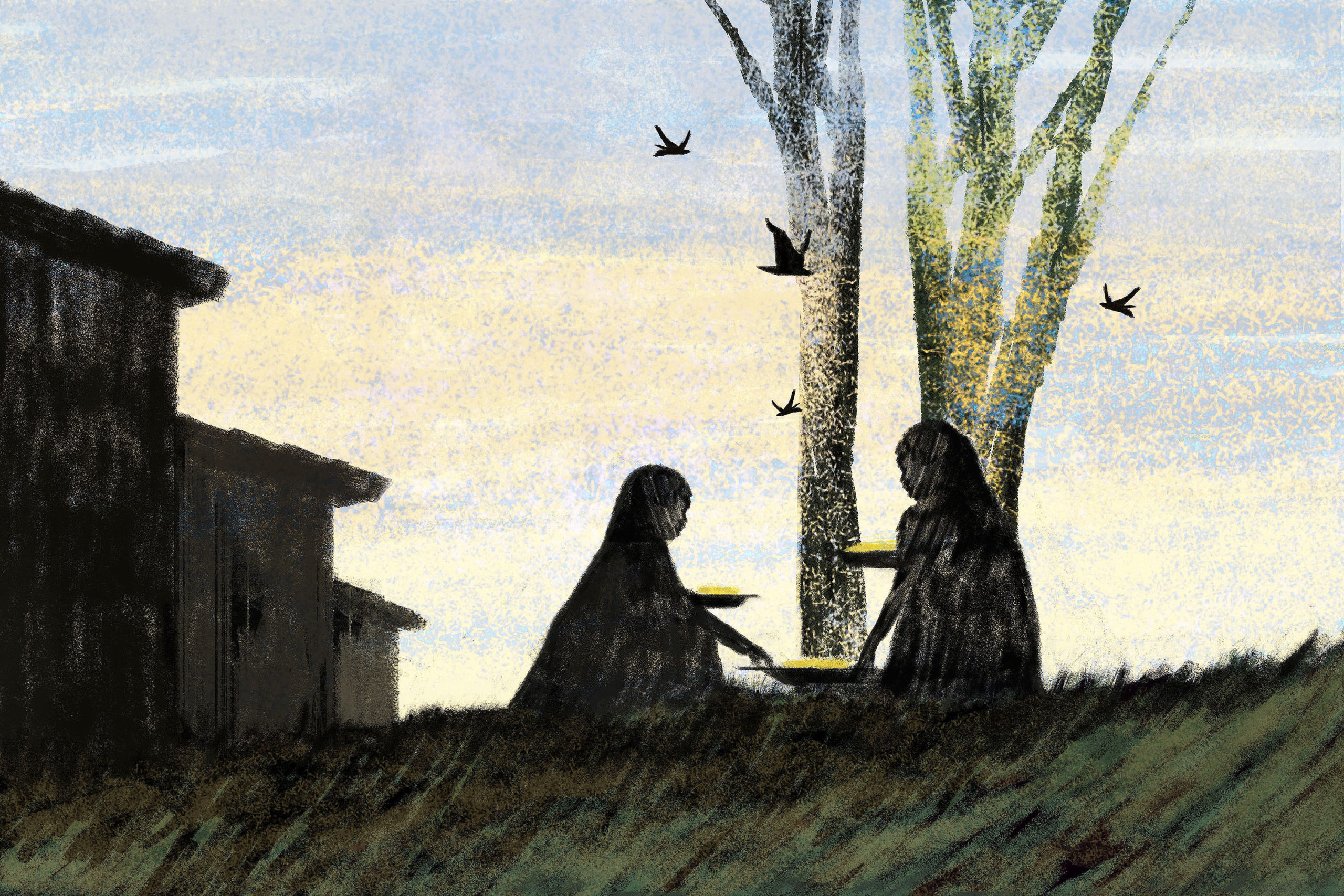This detailed painting showcases a serene, somewhat fuzzy scene that conveys a primitive, impressionistic charm. The sky features a dotted blend of periwinkle blue and cream shades with horizontal streaks of yellow, contributing to a dreamy atmosphere. In the center, two young girls with long hair are crouched or seated in what appears to be a partially grassy, partially fieldlike area, colored in a mix of green, black, and brown hues.

The girls are depicted with simple black and white outlines, engaged in what looks like an activity related to food or cooking. Each holds a black plate or bowl with a yellow substance, while a larger black platter brimming with the same yellow content sits between them on the ground. Their indistinct attire and features underscore the painting's blurred and uncrisp style.

Around them, four black-outlined birds fly, adding a sense of movement to the tranquil setting. Behind the girls, there is a pair of leafless, trunk-and-branch trees that extend out of the frame. To the left, a multi-tiered building resembling a rough sketch of three houses stands, one story, two stories, and three stories high, in shades transitioning from black to dark gray to light gray. The entire composition, from the lush, blowing grass to the ethereal sky, exhibits a hazy, grainy quality, enveloping the viewer in its simplistic yet evocative warmth.